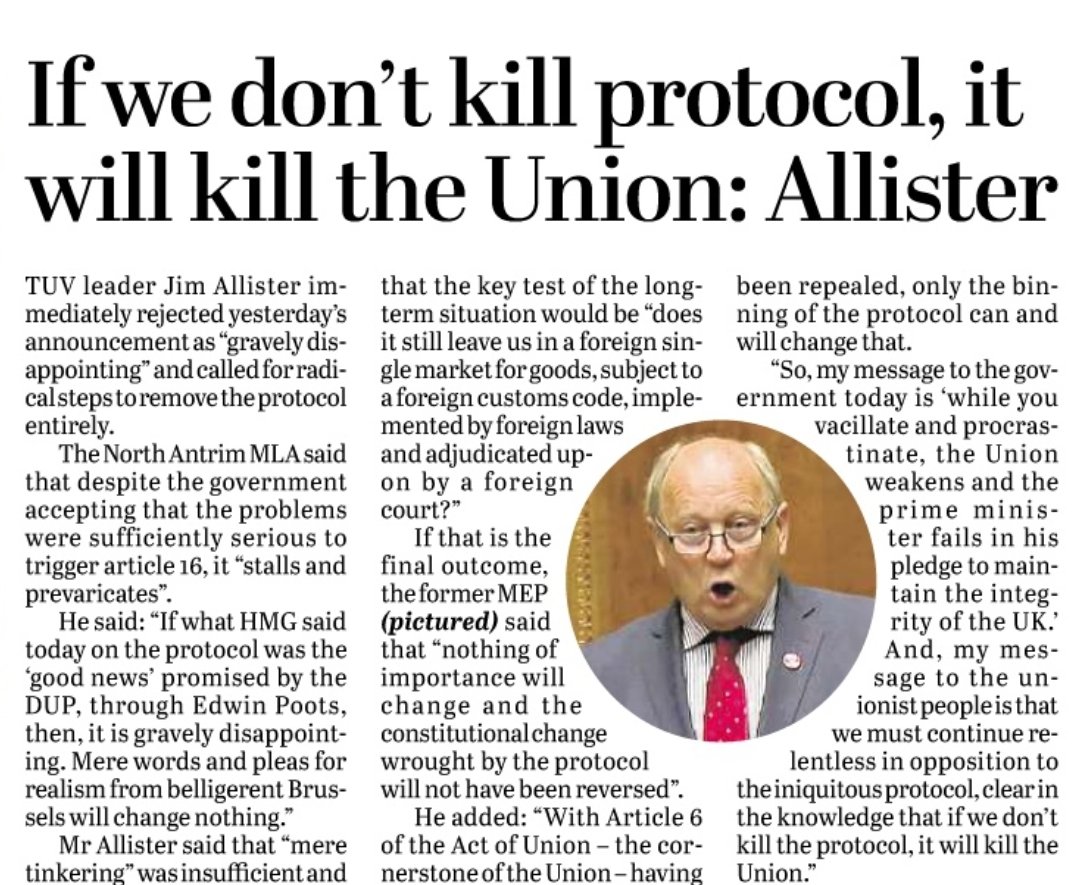The image accompanying the article prominently features an older man at the center, wearing a gray suit, a white shirt, and a striking red tie. His expression is one of surprise, mouth agape, capturing a moment of intense emotion. He is balding and wears glasses, adding a distinguished yet earnest look to his demeanor. 

In bold font, the headline reads: "If we don't kill protocol, it will kill the union – Alistair." Beneath the headline, the body text is presented in a less bold black font, detailing a strong statement by TUV leader Jim Alistair. He vehemently rejected a recent announcement, describing it as "grievously disappointing" and called for radical steps to completely remove the protocol. 

Alistair, a North Interim MLA, criticized the government's stalling and prevarication despite acknowledging the seriousness of the issues which could trigger Article 16. He expressed deep dissatisfaction with the government's response, describing it as empty promises that would do nothing to address the real concerns. 

Alistair emphasized that any mere tinkering with the protocol would be insufficient. He questioned the long-term impact, expressing concerns about remaining subject to foreign markets, customs codes, laws, and courts. Alistair warned that unless significant changes are made, the constitutional impact of the protocol would remain unchallenged. 

He stressed that Article Six of the Act of the Union, a cornerstone of the union, was repealed by the protocol and must be restored. Concluding his message, Alistair warned that if the protocol is not eliminated, it would weaken the union and undermine the UK’s integrity. He rallied unionist supporters to oppose the protocol relentlessly, asserting with urgency: "If we do not kill the protocol, it will kill the union."